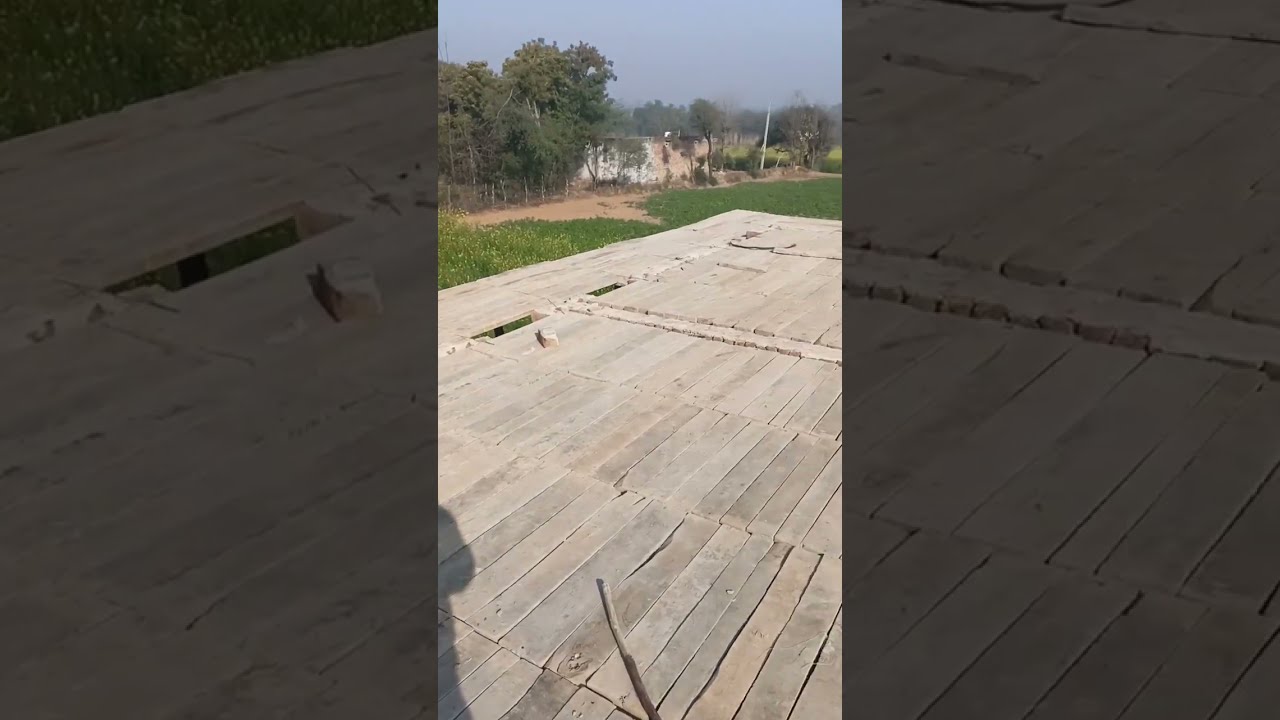The image captures an aged, partly damaged wooden deck, made of light wooden planks, which might be either under construction or in disrepair. The photograph is taken from the perspective of someone standing on the deck, and the viewer can see the shadow of this person. The deck features two missing planks roughly halfway across its expanse. A stick lies diagonally on the deck surface, adding to the scene's rustic ambiance.

In the background, the scene unfolds into a rural landscape with lush green grass fields, a scattering of trees, and an indistinct structure that resembles a shelter or a house to the far left. Additionally, a fence is visible in the distance, further emphasizing the spacious outdoor setting. The sky is a gradient of blue, partially clouded, illuminating the image with daylight. The combined elements create a portrayal of a serene, countryside moment, seen through the lens of someone standing on a weathered deck.